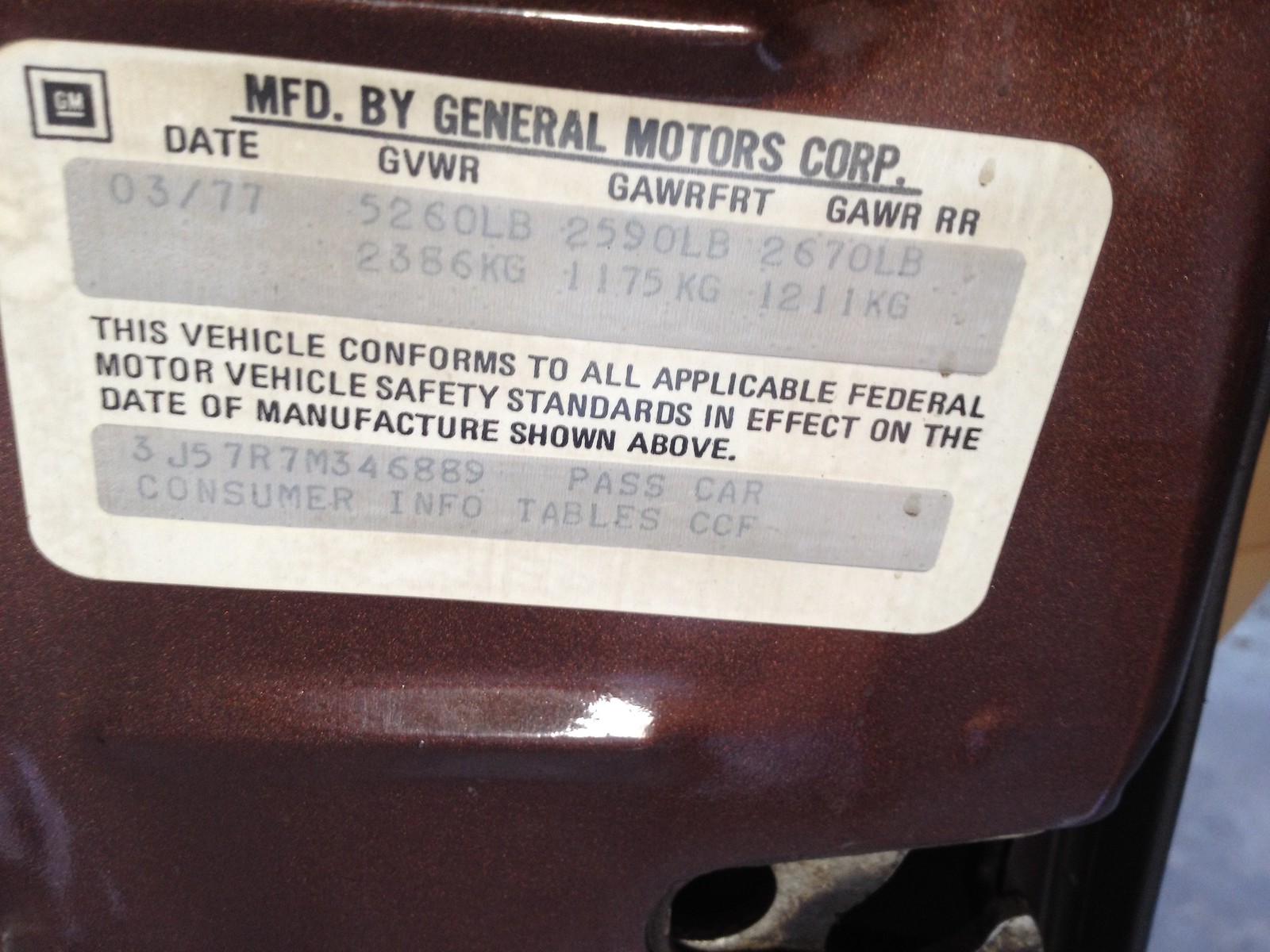This photograph showcases a close-up of a white, rectangular sticker with curved corners affixed to a shiny, maroon-colored metallic surface, likely the inner part of a car door. The prominently displayed sticker features black text. At the top left, the text reads "GM," followed by "MFD by General Motors Corp" in bold. Below this, numbers indicate a manufacture date of "3/77." Further down, the sticker lists automotive specifications including "GVWR," "GAWR FRT," and "GAWR RR" along with corresponding numerical data. A paragraph beneath these details states, "This vehicle conforms to all applicable Federal Motor Vehicle Safety Standards in effect on the date of manufacture shown above." The label also mentions consumer information tables (CCF). This combination of details provides crucial information confirming the vehicle's compliance with federal safety standards at the time of its manufacture.